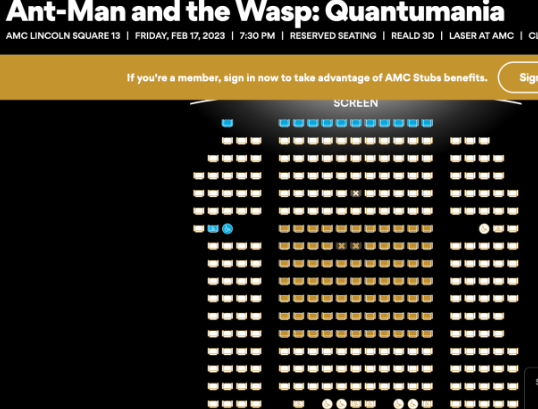This image features promotional details for the movie "Ant-Man and the Wasp: Quantumania" at AMC Lincoln Square. The scheduled showtime is on Friday, February 17th, 2023, starting at 7:30 PM. The screening includes reserved seating in Real D 3D format, enhanced by AMC's Lazer technology. AMC encourages members to sign in to take advantage of exclusive TAUBS benefits. The visual design prominently displays vibrant black, white, yellow, and blue colors.